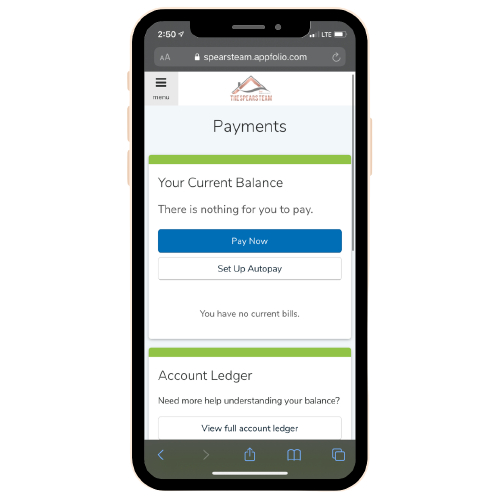The image depicts a vertically-oriented mobile phone set against a stark white background, showcasing an array of information on its screen. The phone features a sleek black bezel with smoothly rounded corners. At the top left corner of the screen, a dark grey header displays the figure "250" accompanied by an upward-pointing arrow. Adjacent to this, on the top right, two out of four white bars signify the mobile data signal strength next to a white "LTE" text box and a predominantly full battery icon.

Directly underneath the header is a URL bar. On its left side, it has a small and a large capital "A" icon, and an adjacent white lock icon, followed by the text "spearsteam.appfolio.com" in white letters. Positioned on the right side of the URL bar is a rounded light grey arrow icon pointing to the right.

The webpage itself begins with a light grey square in the top left corner containing three dark grey horizontal lines stacked vertically, with "menu" written in dark grey below it. To the right of this, a white header displays a logo resembling an orange boomerang with an upward-facing point and a horizontal grey "S" shape. Underneath the logo, there is some blurred orange text.

The main content of the page features a light blue background entitled "Payments." A section beneath this heading contains a green stripe at its top, leading into a white area that declares, "Your current balance: there is nothing for you to pay" in dark text. Below this statement are two buttons: a blue button with "Pay Now" written in white, and a white button outlined in light grey with "Setup Auto Pay" in black text. At the bottom of this section, a thin line of small text reads, "You have no current bills."